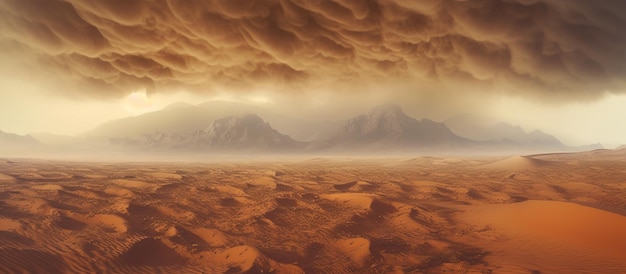This image, likely AI-generated, depicts an eerie and surreal desert landscape with a windy ambiance. Orange sand forms the foreground, characterized by small, dune-like mounds and gently rolling hills, creating a texture reminiscent of moon craters upon first glance. In the background, the closest visible layer features rugged, gray-brown mountains, behind which faint silhouettes of a larger mountain range can be discerned through a thick hazy atmosphere, possibly caused by a sandstorm or distant rain.

Dark, tumultuous clouds dominate the sky, lending a heavy and foreboding feeling to the scene. Although these clouds suggest an impending storm, there is no visible rainfall in the image itself. The clouds display a mesmerizing complexity, appearing fluffy in some areas while forming flat, ominous stretches in others. Subtle streaks of yellow, which could be the remnants of lightning, add to the surreal quality, casting an otherworldly glow over the landscape. Overall, the interplay of dynamic natural elements creates a dramatic and otherworldly visual experience.